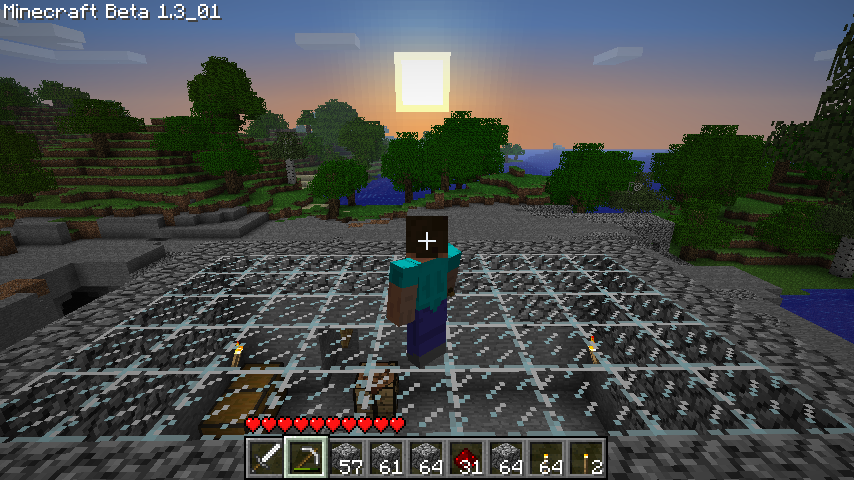This screen capture from the game Minecraft Beta 1.3_01, displayed in landscape mode, features an iconic pixelated scene. At the very top left corner of the screen, the version of the game, "Minecraft beta 1.3_01," is clearly indicated. Prominently in the center, there's a human-like character with a distinctly blocky, Lego-like appearance. The character is adorned with a green shirt, brown arms, and blue pants. Though the character's feet are indistinct, a gray section appears where the feet would typically be. Superimposed right over the character's torso is a black square with a white cross, likely indicating the player's cursor or targeting mechanism. At the bottom of the screen, there is a series of gray squares, probably part of the game's interface or inventory system. The first square features a diagonal slash, with the subsequent squares numbered sequentially, though the exact numbers are not specified. The overall image encapsulates the nostalgic and rudimentary aesthetic of the game's beta version, complete with its simplistic yet charming graphical elements.